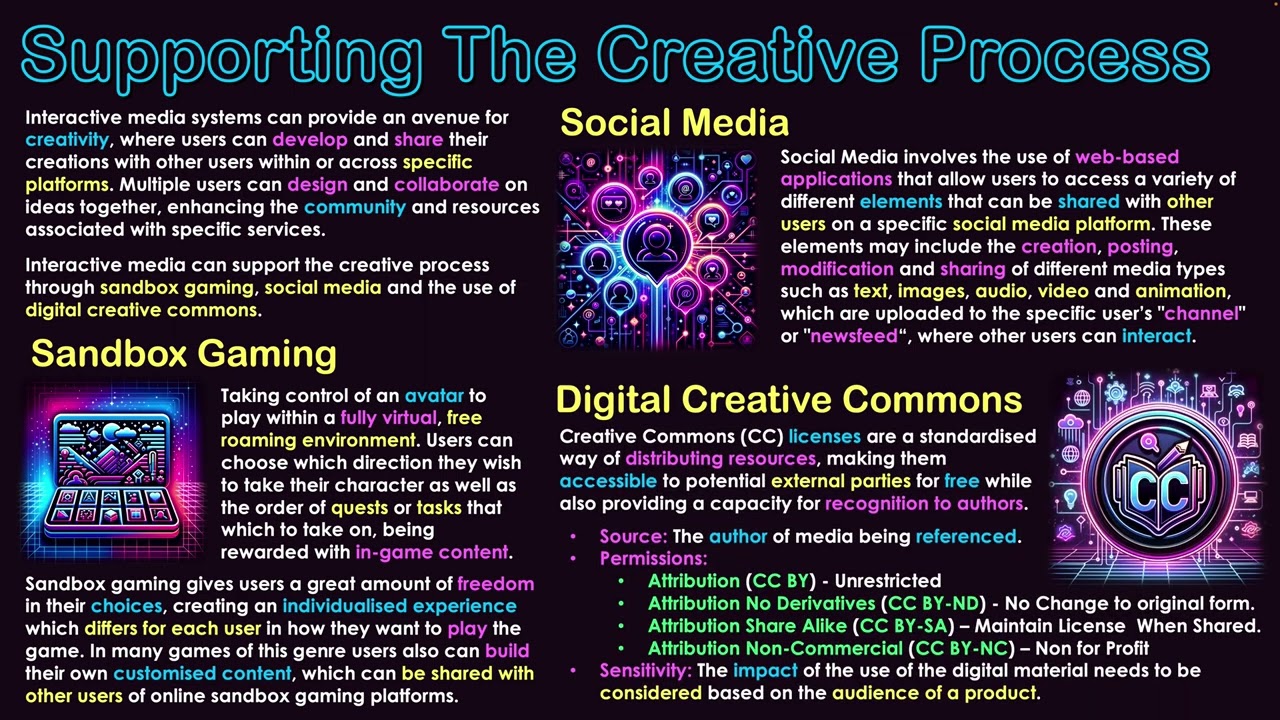The image features a predominantly black background with text and visuals highlighting various aspects of the creative process. At the top, in a combination of upper and lower case letters outlined in blue, it reads "Supporting the Creative Process." The main content is divided into two sections: on the left, a series of detailed paragraphs and on the right, three categorized sections each with descriptive explanations.

On the left, white text begins with "Interactive media systems can provide an avenue for," followed by the word "creativity" in blue. Additional colored text emphasizes key concepts: "Develop and share" in purple, and "specific platforms" in yellow. The text explains that multiple users can "design and collaborate" (purple) on ideas together, enhancing "community" (blue) and resources associated with specific services.

To the right, three key areas are highlighted in yellow: "Sandbox Gaming," "Social Media," and "Digital Creative Commons." Each section includes detailed explanations, where "Sandbox Gaming" and "Social Media" are described individually, and "Digital Creative Commons" further breaks down into bullet points in green text.

Accompanying the text are three images, possibly representing a laptop or computer, rendered in shades of purple, black, and pink, adding a visual element to the presentation. The overall layout and color-coded text indicate this image serves as an infographic promoting and explaining different interactive media systems and their role in fostering creativity.